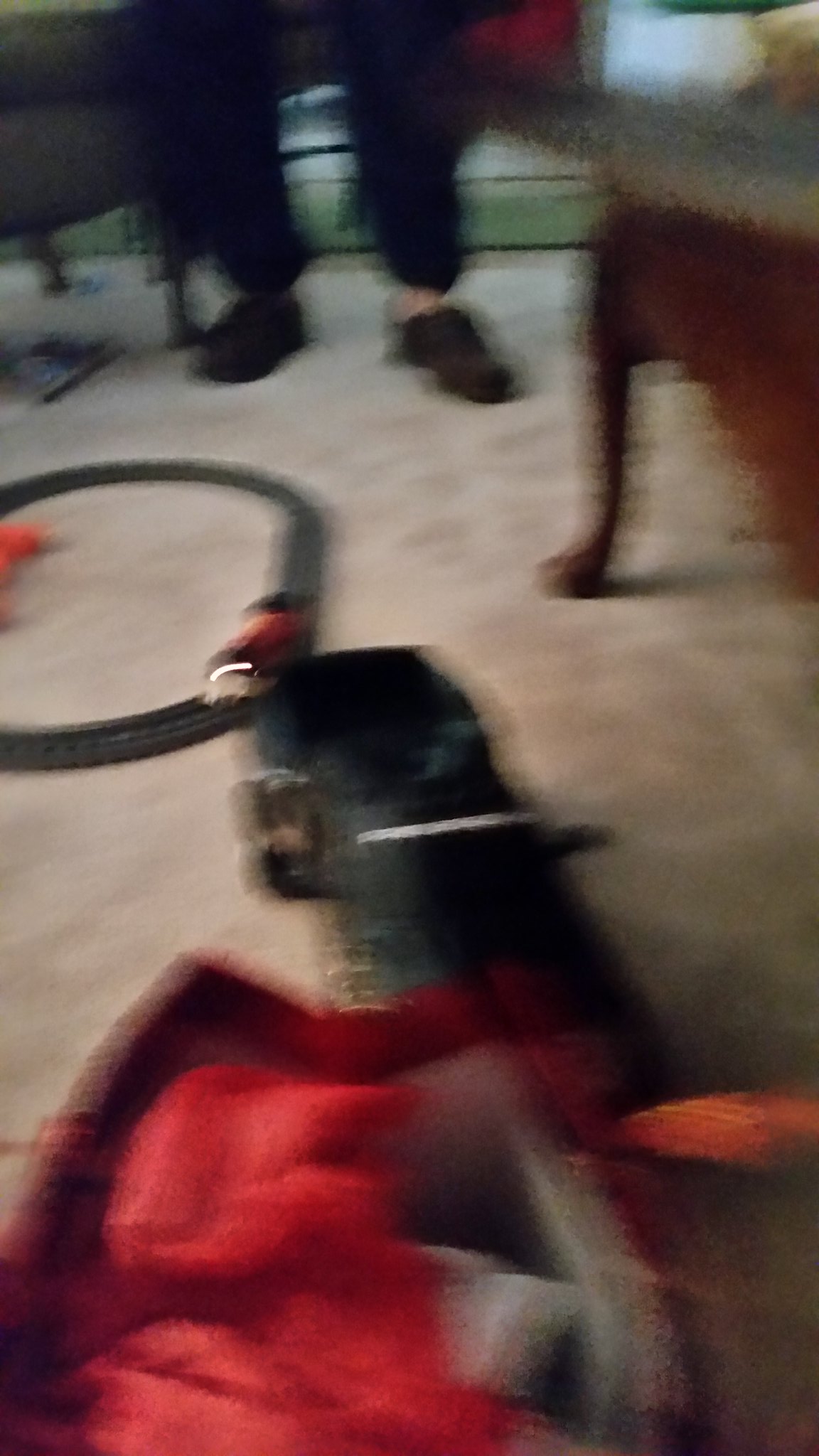A very blurry image captures the interior of a house, with the camera pointed towards the floor. In the foreground, a black object of undetermined nature is present. Positioned in front of it is a bunched-up red material, adding a splash of color to the scene. Behind this, there's an oval-shaped object resembling a miniature train track with a red railroad engine and some black and white highlights navigating the track.

The background reveals a partial view of a person, cropped at the top, seated. The individual is wearing dark pants and dark shoes, with either no socks or tan-colored socks. One can also see the leg of a wooden chair, covered with gray fabric. The floor is carpeted in beige, adding a subtle, neutral backdrop to the composition.